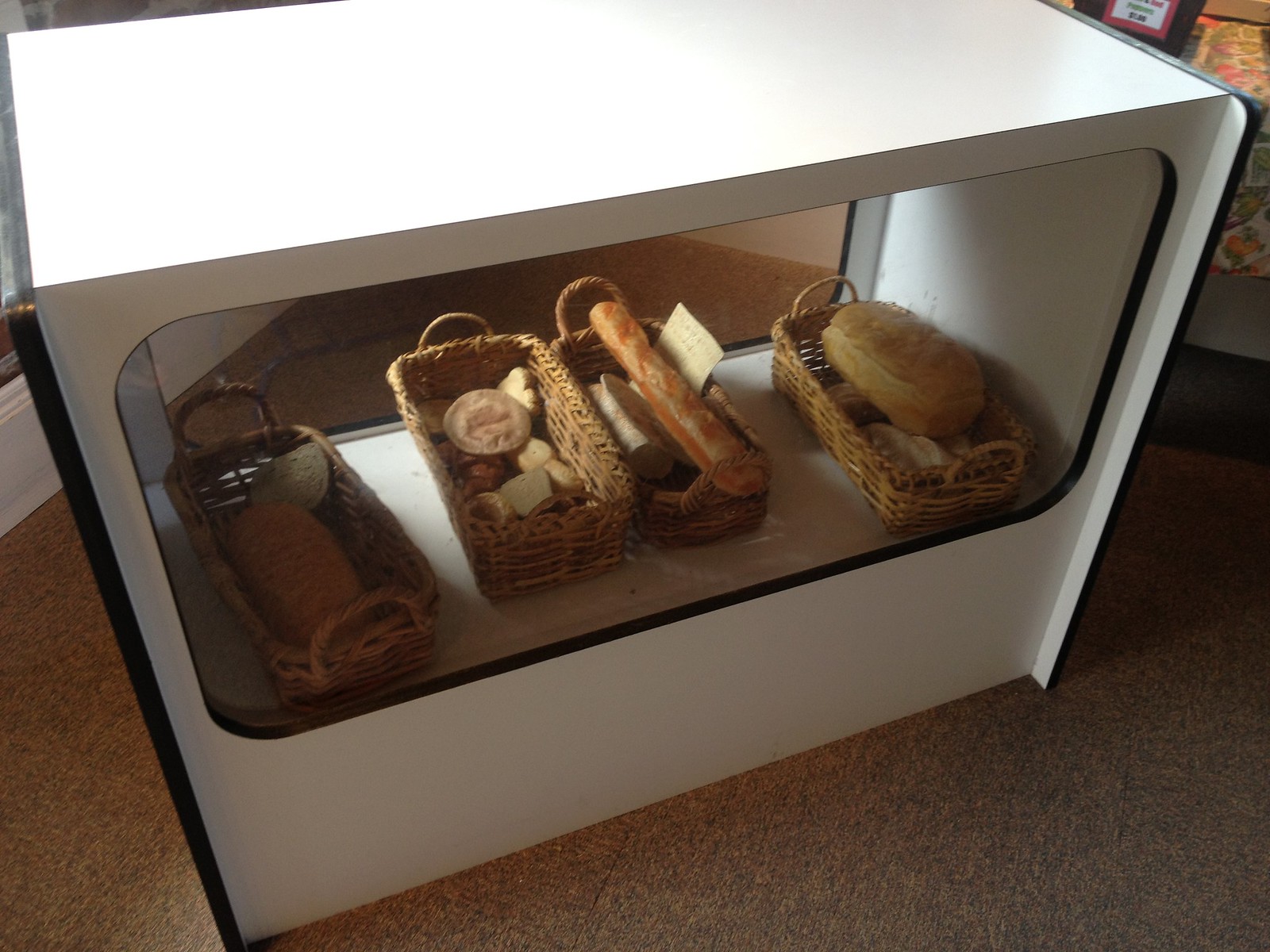The image is a color photograph depicting a detailed display on a white, compartmentalized countertop with a light tannish-colored ground below. The compartment is sectioned into four wicker baskets, each containing different types of bread and covered with clear, see-through rectangular covers. 

On the right side, there is a larger oval loaf of bread. Adjacent to it, towards the center, is a basket with thinner, light brown baguettes and a small piece of pastry at the top. The basket next to it has a long loaf stretching from one side to the other with a note leaning against it. Finally, the basket on the left, which is partly obscured by shadows, contains a shorter loaf and a few smaller pieces of bread. The baskets are all equipped with handles on either side. The white container housing these baskets has black outlines along the sides, resembling a large bread box.